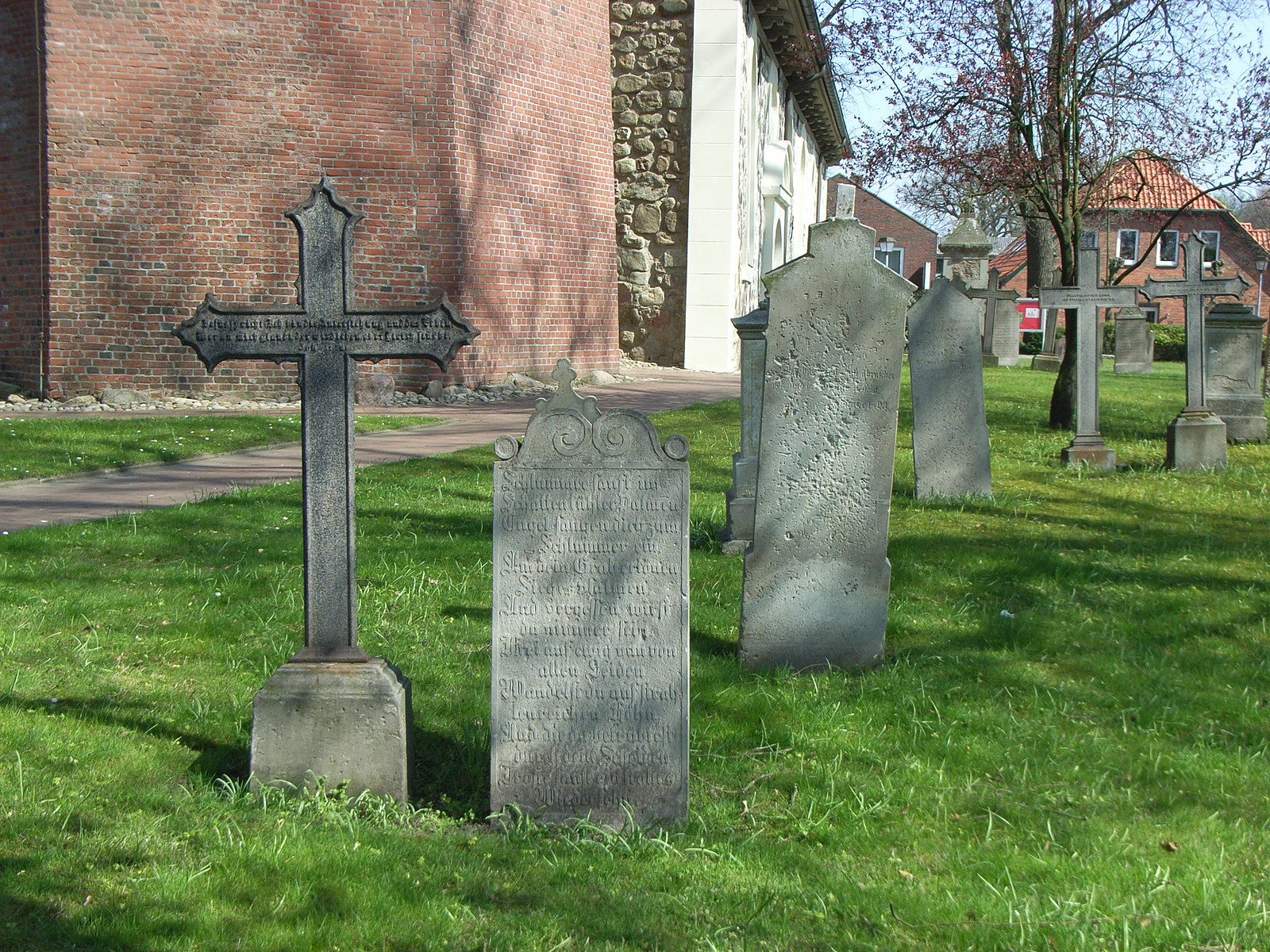This photograph captures an old cemetery on a flat grassy lot. Prominently, there are various headstones, including several tall, narrow tombstones and crosses rising from stone pedestals. The stones themselves are aged and weathered, with some engraved text that has faded over time, rendering it illegible. Notably, there's a cross to the left, also mounted on a pedestal, and to its right, more traditional tombstones with rounded tops. Beyond these, there are additional cross-shaped headstones set further back, some featuring intricate designs that deviate from the typical rounded shapes.

Behind the first cross is a pathway leading towards an older, sturdy brick building. Further to the right, there's an additional building that’s harder to discern in detail. The cemetery is surrounded by green grass, indicating an outdoor setting, and appears to be captured in fall due to the bare trees visible in the background. The buildings extending into the distance include a brick house with a terracotta tile roof, enhancing the historical ambiance of this tranquil resting place.